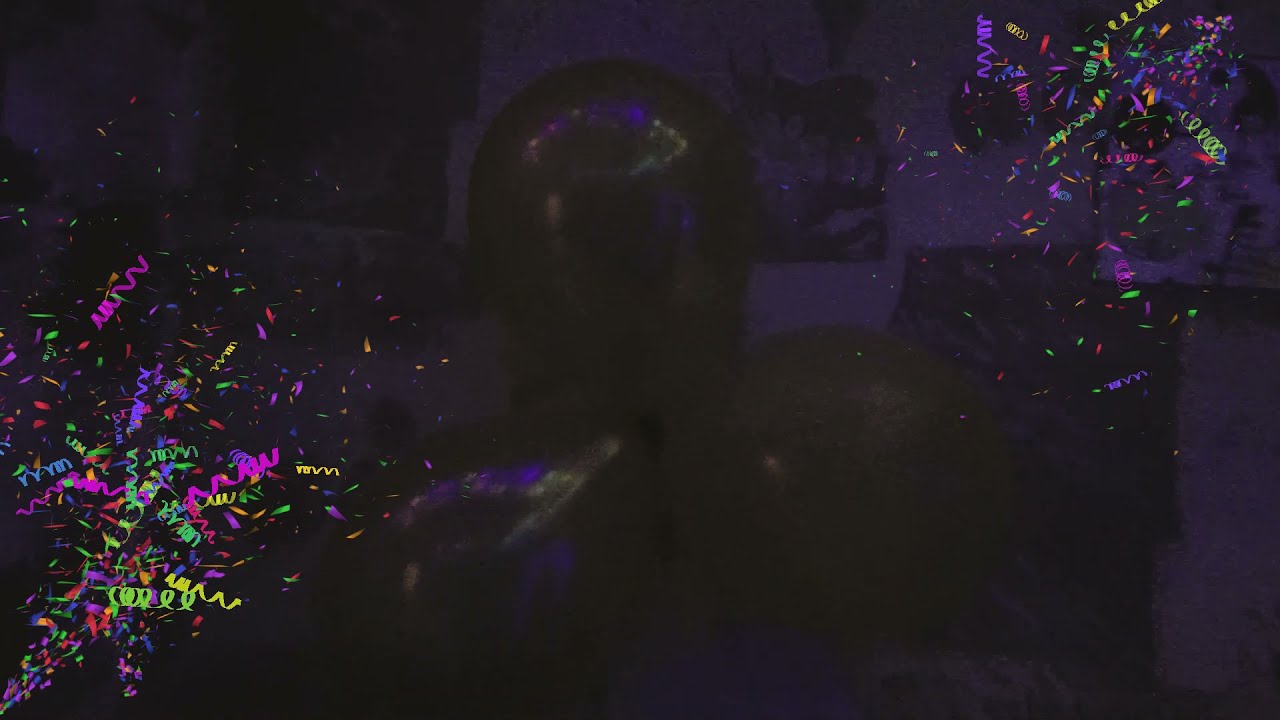The image depicts a dark, abstract scene with faint purple hues overlaid across the background. At the center, there is a barely discernible outline of a person or possibly three balloons tied together, framed against a wall that features a vague poster or doorway, giving a sense of a dimly lit room. In the lower left and upper right corners, there are bright, digitally-added confetti and streamers in a variety of colors, including blue, red, green, purple, yellow, and pink. These festive elements appear to be strategically placed, with the bottom left corner exhibiting a more prominent burst of confetti that streams upwards, contrasting with the top right corner's subtler display. Despite the overexposed nature making much of the background and central figure obscure, the lively, vibrant confetti stands out, creating an interesting juxtaposition against the predominantly dark and shadowy environment.